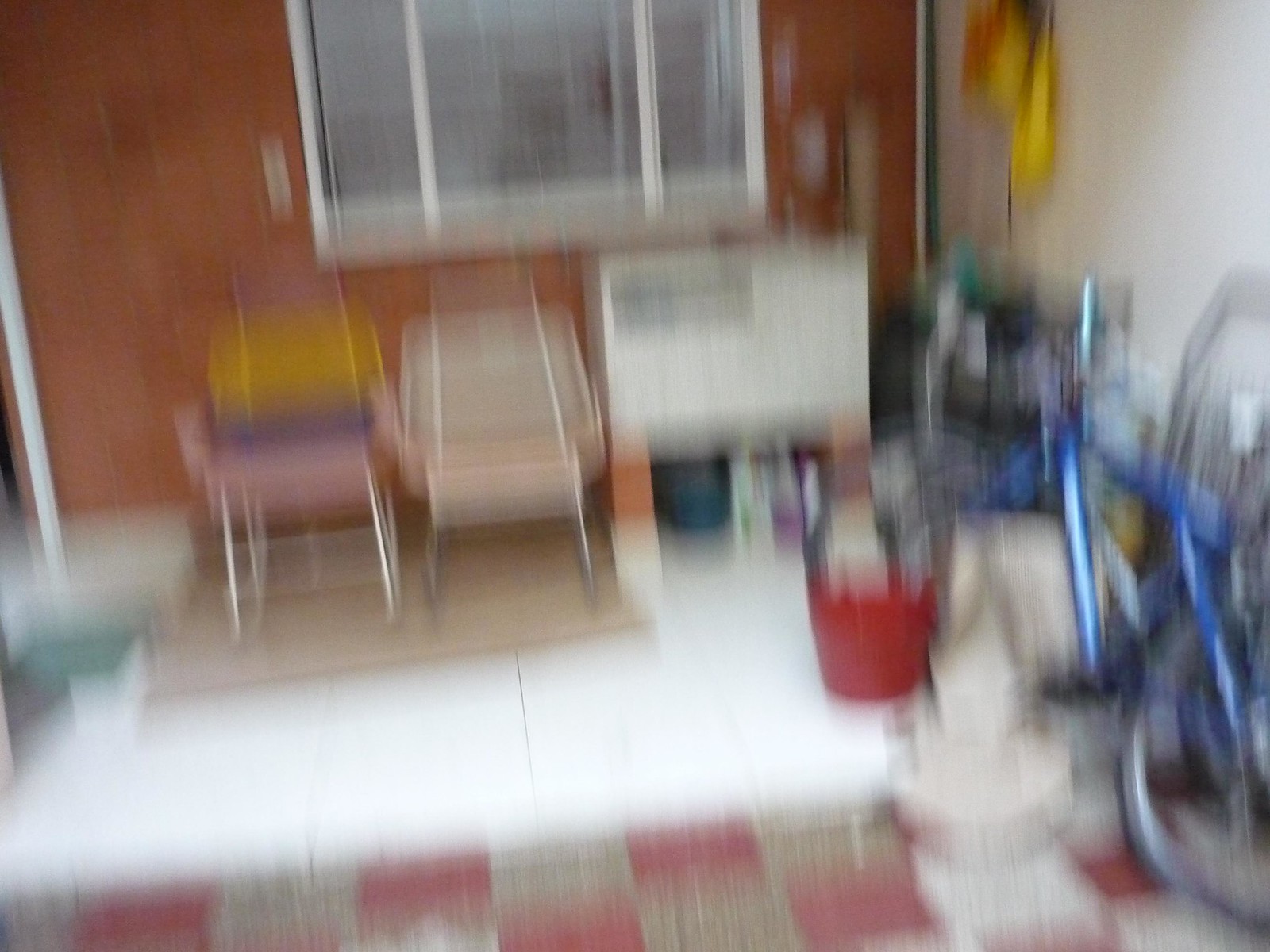In this slightly blurry image of what appears to be a classroom or workshop, the background features a burnt orange wall adorned with a white sliding window. Positioned in front of the wall are modern, multi-colored chairs with sleek metal legs; one chair stands out with its vibrant yellow, purple, and pink hues, while the other has a more muted ivory tone. Beside the chairs sits a square chest on wooden legs, resting on a patch of white spray-painted flooring. Dominating the foreground is a distinct red and white checkered floor pattern. On the right side of the frame, a white wall displays what seems to be yellow work clothes or an apron hanging up. Nearby, several bike parts, including a bike frame and a red bucket, are visible, adding to the eclectic mix of items in the space.